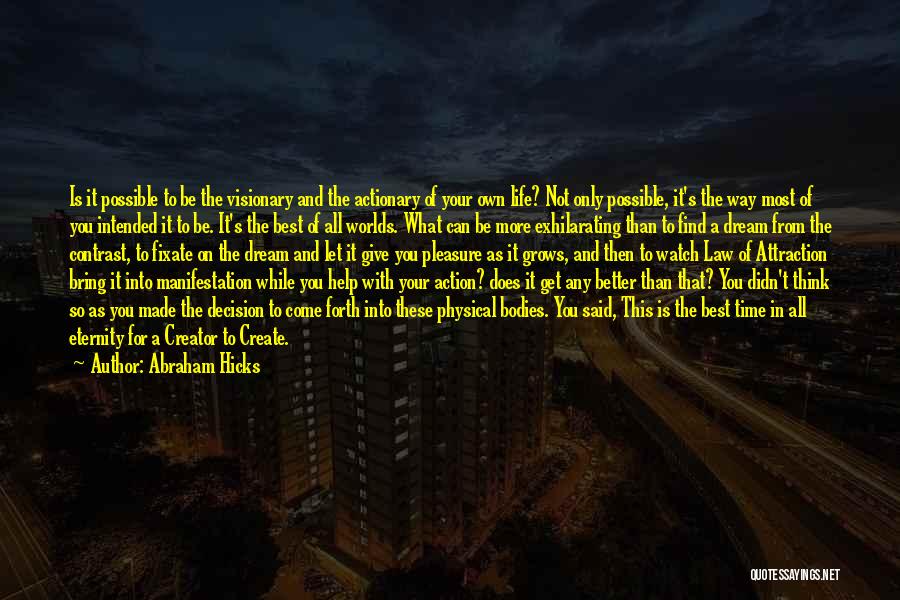The image features a prominent quote in yellow text against the backdrop of a nighttime cityscape. Appearing like a paragraph of words, the text reads: "Is it possible to be the visionary and the actionary of your own life? Not only possible, it's the way most of you intend it to be. It's the best of all worlds. What can be more exhilarating than to find a dream from the contrast? To fixate on a dream and let it give you pleasure as it grows. And then to watch the law of attraction bring it into manifestation while you help with your action. Does it get any better than that? You didn't think so as you made a decision to come forth into these physical bodies. You said, this is the best time in all eternity for a creator to create." The quote is attributed to Abraham Hicks and is centered in the image.

The background reveals a dark, dimly lit nighttime cityscape. On the left, several tall buildings stand with a combination of black and brown facades dotted with windows in various shades of gray and silver. On the right side, there's a flyover with street lights illuminating light trails below, suggesting movement. The sky above is a blend of dark blue and black, interspersed with black clouds. Beneath the quote and to the right, in white text, it says "quotes.saying.net," indicating the source of the image. This detailed description encapsulates both the inspiring words and the vivid nocturnal urban setting.